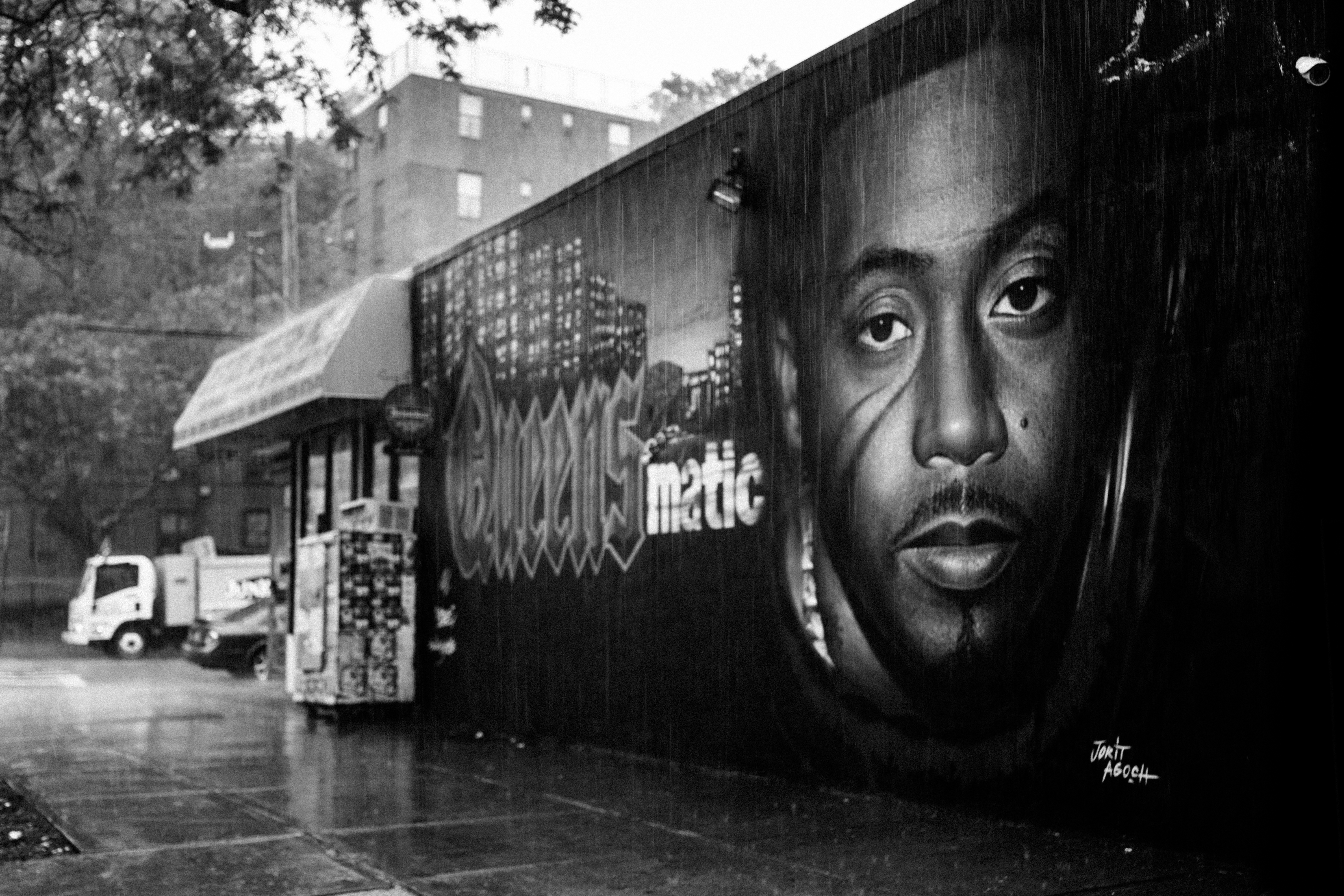The photograph captures a detailed black-and-white image of a mural painted on the side of a business located in a bustling downtown urban area. The mural is prominently displayed on the right side of the image and spans the entire height of the building. It features a serious-faced portrait of Nas, the rapper, easily identifiable by his distinctive facial features, including his black hair, beard, and mustache. Adorning the mural, in large text, are the words "Queen's Matic" set against a painted cityscape with illuminated windows of multiple square buildings. Adjacent to the mural, the entrance to what appears to be a convenience store or small grocery store is visible, complete with an ice machine and an overhang extending above the doorway. The bottom-left section of the image reveals a pedestrian walkway made up of large concrete tile sections, extending towards a road visible in the middle far section, where a truck and the back end of a parked car can be seen. The lower right-hand corner of the mural contains the artist's signature, possibly reading "Jory" or "Jort Agok." The overall scene is enhanced by the presence of a nearby tree and a multi-story building in the background, contributing to the urban atmosphere depicted in this street artwork.